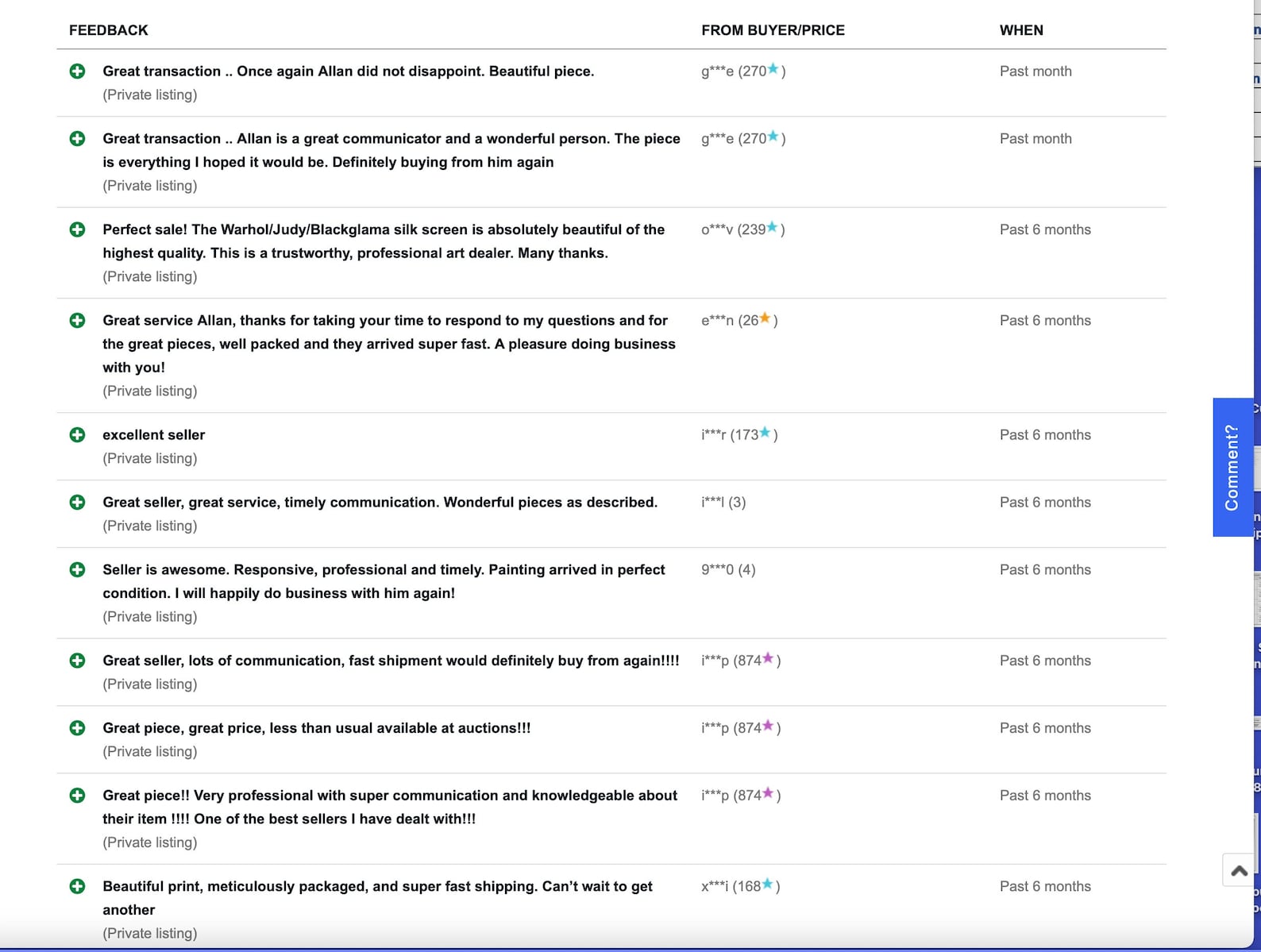**Caption:**

A color image displaying a detailed eBay feedback page against a white background. At the top of the image, the word "Feedback" is prominently displayed. Below this header, there are several bolded sentences, each accompanying a small round green circle on the left side. The image shows various user reviews, with usernames, ratings, and stars, typical of eBay's feedback section. The usernames include small asterisks, a common feature for privacy on eBay.

On the right side of the page, there are columns labeled "Past Month" and "Past Six Months." The feedback comments are overwhelmingly positive, praising a seller named Alan. Phrases such as "great transaction," "excellent seller," and "perfect sale" are frequently mentioned. Specific feedback includes praise for Alan's communication skills, the high quality of items sold, and timely shipping. One notable review describes a Warhol Judy black silkscreen as "absolutely beautiful" and of the "highest quality." Another comment highlights Alan's professionalism as an art dealer.

Overall, the feedback page reflects Alan as a highly respected and trustworthy seller, consistently providing exceptional service and high-quality art pieces, as evidenced by numerous satisfied buyers.